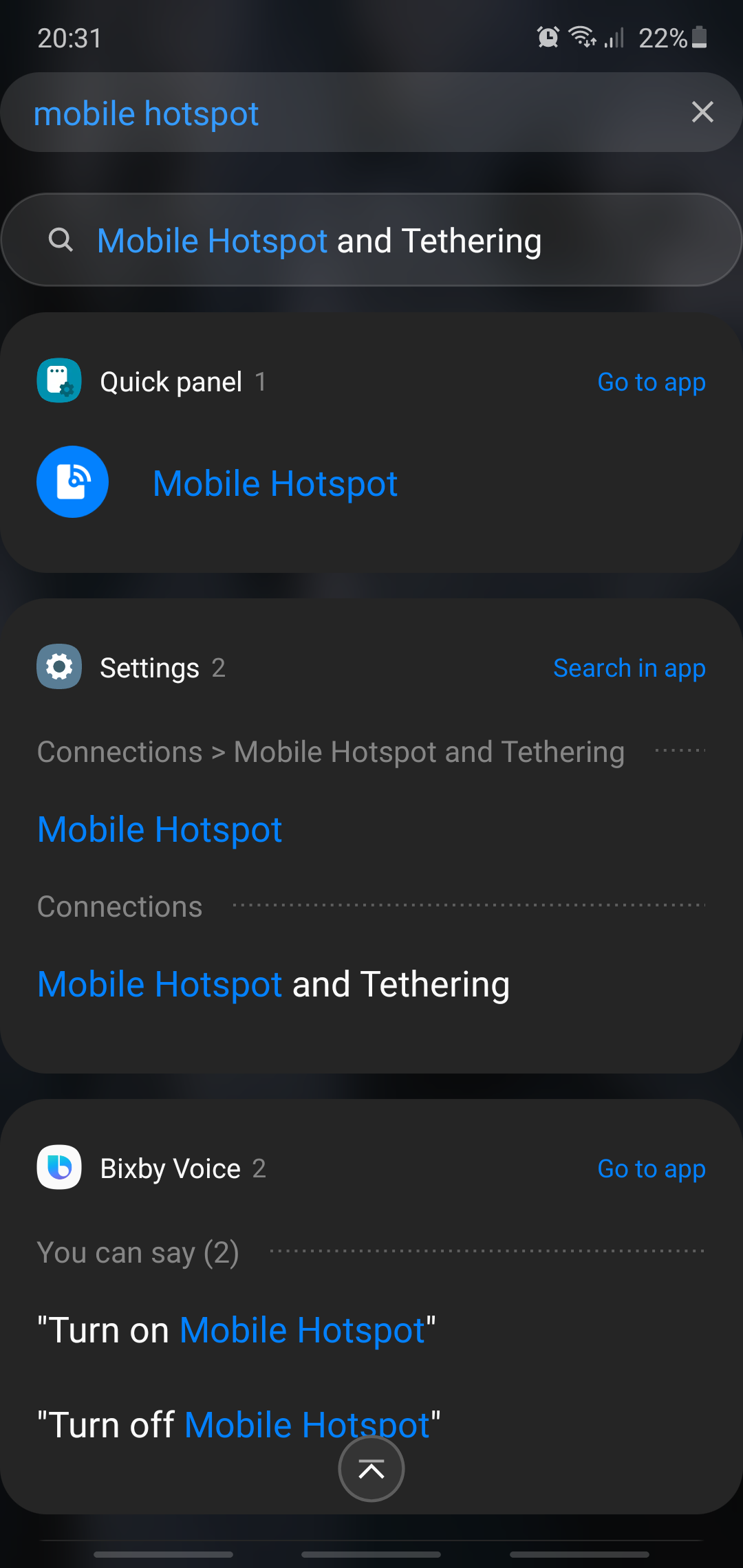A phone screenshot with a black background displaying the time as "20:31" on the top left. The top right shows a row of icons: a clock, a Wi-Fi signal, a signal strength bar showing two out of four bars, a battery percentage at 22%, and a battery icon indicating the same. Below these icons is a gray oval search input labeled "mobile hotspots" in blue text, with a light gray 'X' on the far right.

Further down is another oval containing a search icon and the text "mobile hotspot" in blue and "tethering" in white. Below this, there is a large oval with "Quick Panel" in white text, followed by a number one in gray. To the right, it shows "Go to app" in blue text next to a blue icon labeled "mobile hotspot."

Below this section, several settings options appear: 
- "Connections" leading to "mobile hotspot" and "tethering" in gray text.
- "Mobile hotspot" in blue text, followed by "connections" in gray, and "mobile hotspot" in blue again.
- "Tethering" in white text.

Lastly, the text indicates "Bixby Voice," followed by "Go to app" in blue text with "2" in gray text in parentheses. Suggested voice commands like "turn on mobile hotspot" and "turn off mobile hotspot" are marked in quotation marks.